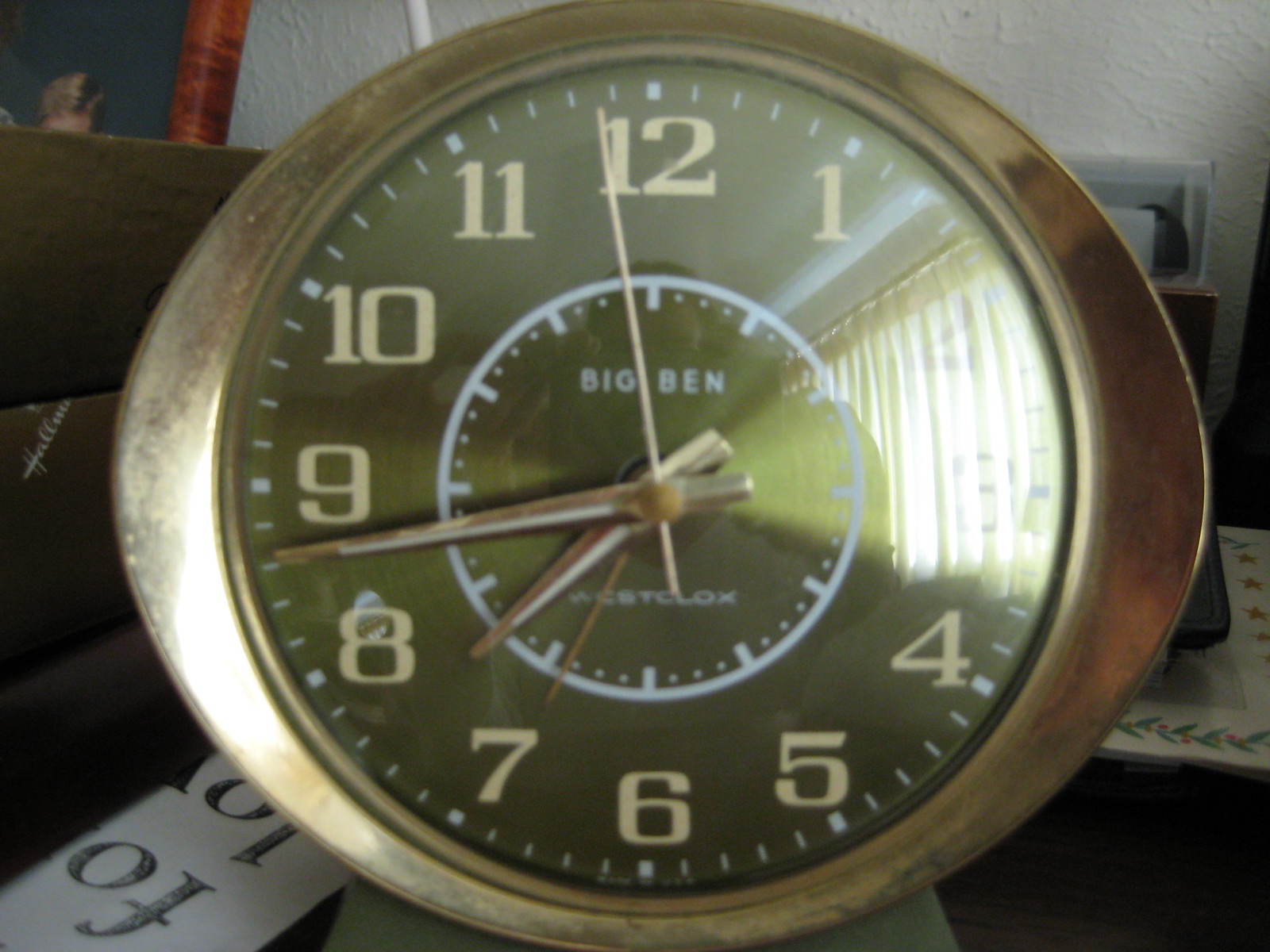This is a close-up image of a retro-styled alarm clock resting on a wooden desk. The clock features a distinctive eye-shaped, silver frame with a black face adorned with beige Arabic numerals marking each hour. At the center of the clock, there’s a smaller, white second clock face with needle-shaped hour, minute, and second hands, all in a matching silvery chrome color. The time displayed is 7:38, with the second hand on the 59th second. The desk, made of wood, is positioned next to a wooden headboard. In the background, there are gray, textured plaster walls adorned with a family photo where a young boy's head is visible. Additional items on the desk include a computer, a doily, and a book, adding to the scene's homely ambiance.